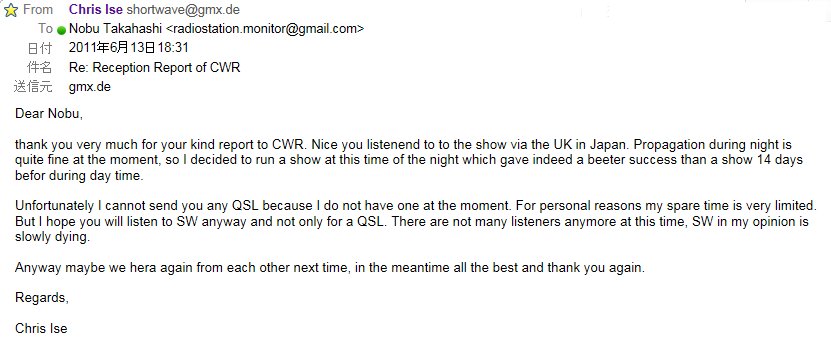The image is a screenshot of an email, left aligned against a solid white background. The email is from Chris Eyes, using the address chrisiceshortwave@gmx.de, to Nobu Takahashi at radiostation.monitor@gmail.com. The email is regarding a reception report for CWR. It begins with, "Dear Nobu, thank you very much for your kind report to CWR. Nice you listened to the show via the UK and Japan. Propagation during night is quite fine at the moment, so I decided to run a show at this time of the night, which indeed had better success than a show 14 days before during daytime. Unfortunately, I cannot send you any QSL because I do not have one at the moment. For personal reasons, my spare time is very limited, but I hope you will listen to SW anyway and not only for a QSL. There are not many listeners anymore at this time. SW, in my opinion, is slowly dying. Anyway, maybe we hear again from each other next time. In the meantime, all the best and thank you again. Regards, Chris Eyes.” The email contains some Japanese characters and there's a yellow star in the upper left-hand corner. The message highlights challenges with the availability of QSL cards, limited listener engagement, and Chris' hope for continued interest in shortwave radio.